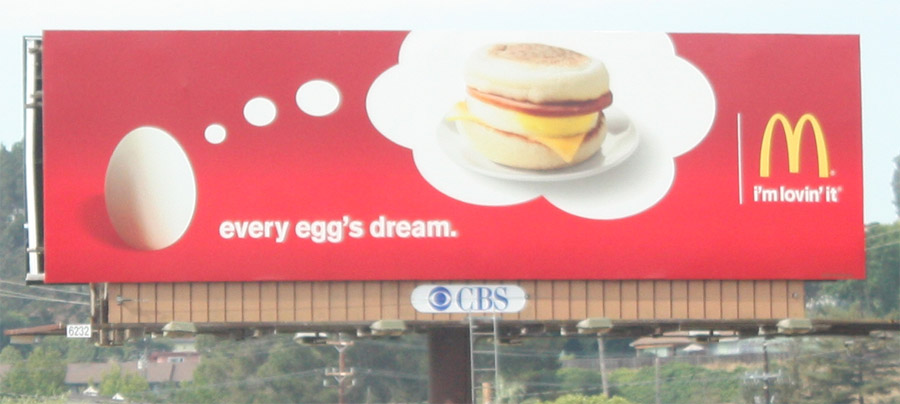The photograph captures a billboard advertisement for McDonald's, specifically promoting the Egg and Ham McMuffin. The background of the billboard is a vibrant red, adding a sense of urgency and excitement to the advertisement. Dominating the center of the billboard is an image of a breakfast egg depicted with a whimsical thought bubble. Inside this thought bubble, the egg is daydreaming about a delicious Egg and Ham McMuffin. This visual is accompanied by the playful caption "Every egg's dream," suggesting that this McMuffin is the pinnacle of breakfast delights.

To the right of the thought bubble, the iconic McDonald's arches are prominently displayed, serving as an unmistakable signature of the brand. Below the arches, the well-known tagline, "I'm lovin' it," is written, reinforcing McDonald's global slogan.

The bottom of the billboard features the CBS logo, indicating that this advertisement might be strategically placed in a high-traffic area for maximum visibility. 

The visual representation of the Egg and Ham McMuffin is detailed and mouth-watering. The sandwich is presented on a simple white dish against a white background, making the vibrant colors of the ingredients stand out. The McMuffin consists of a perfectly toasted English muffin with a delightful slice of fried ham, a neatly rounded egg patty, melted cheese, and topped off with the other half of the English muffin.

Overall, the billboard is a bold, engaging advertisement that effectively highlights the appealing components of the Egg and Ham McMuffin, aiming to entice every passerby to indulge in this McDonald's breakfast classic.